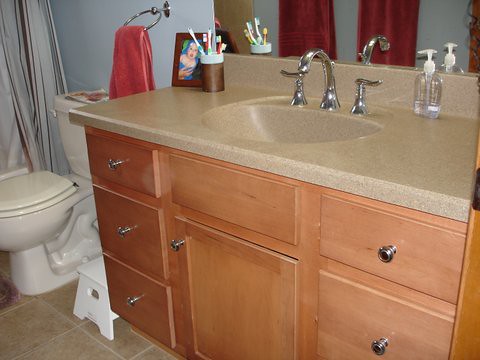The photo captures the interior of a modest bathroom. To the far left, a white toilet occupies the corner next to a bathtub partially hidden by a hanging shower curtain. Adjacent to the toilet, a striking red towel is elegantly draped on a circular wall-mounted ring. A white footstool rests nearby, adding a touch of practicality to the space.

The focal point of the room is the sink area, characterized by a light brown countertop that spans both sides of a centrally-located white sink. The sink is fitted with a standard silver faucet equipped with twin handles. To the right of the sink, a clear plastic soap dispenser with a squeeze trigger is conveniently placed. On the counter's left side, a collection of toothbrushes is neatly arranged beside a photo in a frame.

Above the sink, a large mirror dominates the wall, reflecting the elements of the room. In its reflection, two towels are visible on the opposite wall, providing continuity in the bathroom's decor. Below the counter, functional drawers offer storage space, completing the practical yet cozy atmosphere of this everyday bathroom.